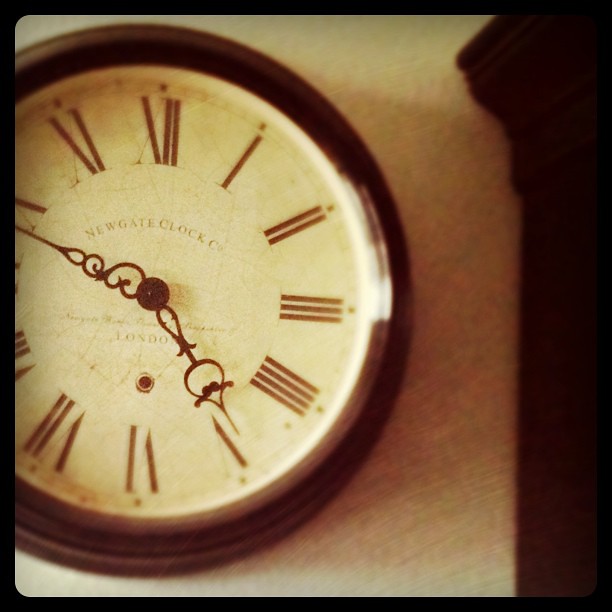The photograph features a vintage-inspired clock mounted on a tan-colored wall, rendered in a sepia tone that lends an old-time artistic feel to the image. The clock is encircled by a black outer border and has a tan face, appearing cream due to the sepia filter. The Roman numerals from 1 to 12 are in black, accompanied by the inscription "Newgate Clock Company, London" prominently displayed on the face. The clock's hour and minute hands are intricately designed with ornate loops, almost forming heart shapes at their tips, and there's no second hand. The time displayed is around 4:48 to 4:49. To the right, a dark wooden banister, possibly the side of a cabinet or shelf, adds to the photo's vintage ambiance with its decorative design.